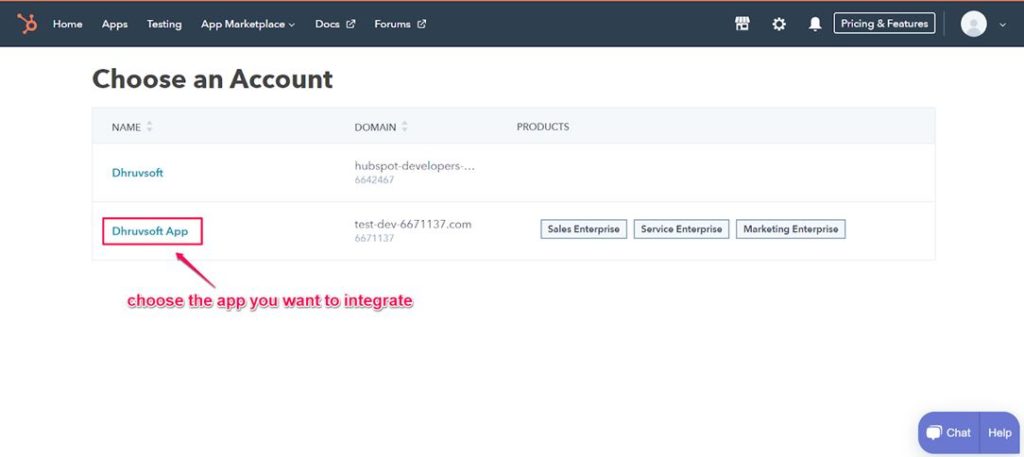**Web Interface Detailed Description:**

At the top of the web interface is a dark black navigation bar featuring several menu items and icons. The menu options displayed in this bar include "Home," "Apps," "Testing," "App Marketplace," "Docs," and "Forums." Adjacent to these menu items are icons for a storefront, settings gear, and notifications, alongside options for "Pricing" and "Features."

Beneath this navigation bar, the interface prompts the user to "Choose an Account." Following this prompt, there are categories for "Name," "Domain," and "Products." For the first account listed, the "Name" is "dhnuvsoft," the "Domain" is "HubSpot Developers," and the "Products" section is currently empty.

Proceeding to the next section, another account named "dhnuvsoft App" is displayed. This section is highlighted with a pink border and features a prompt in pink text stating "Choose the app you want to integrate." Below this, it lists "test develop 667 1137.com" under "Domain." The "Products" field for this account includes "Sales Enterprise," "Service Enterprise," and "Marketing Enterprise."

At the bottom of the interface, there is a purple bar with white text offering additional functionality. This bar includes options for a "Chat" function and a "Help" function.